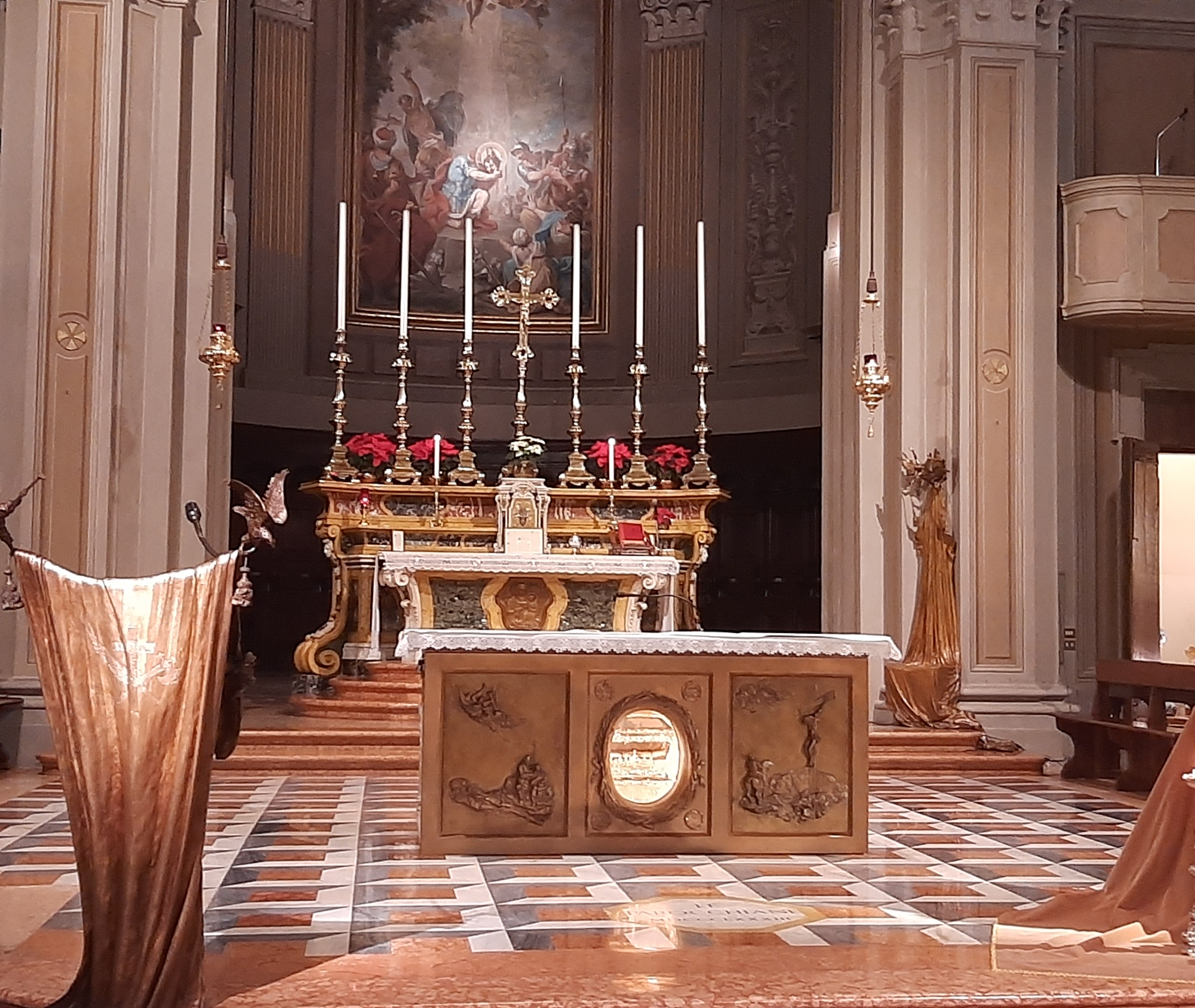The image depicts the main hall of a religious institute, possibly a church, characterized by a grand and ornate design. Central to the scene is an intricately designed wooden podium situated on the left, equipped with a microphone. The foreground features a large, elegant table placed upon a shiny, ornately patterned tile floor. Two columns frame the midground, leading the eye towards steps at the back of the hall. These steps ascend to another smaller, elaborate table adorned with six tall, white candlesticks. Central to the background is a prominently displayed ornate cross, positioned in front of a painting on the wall. The rich color palette includes browns, grays, whites, blues, reds, and blacks, which enhance the grandeur of the setting. The surroundings convey a sense of solemnity and reverence, characteristic of a religious space designed for sermons or special ceremonies.